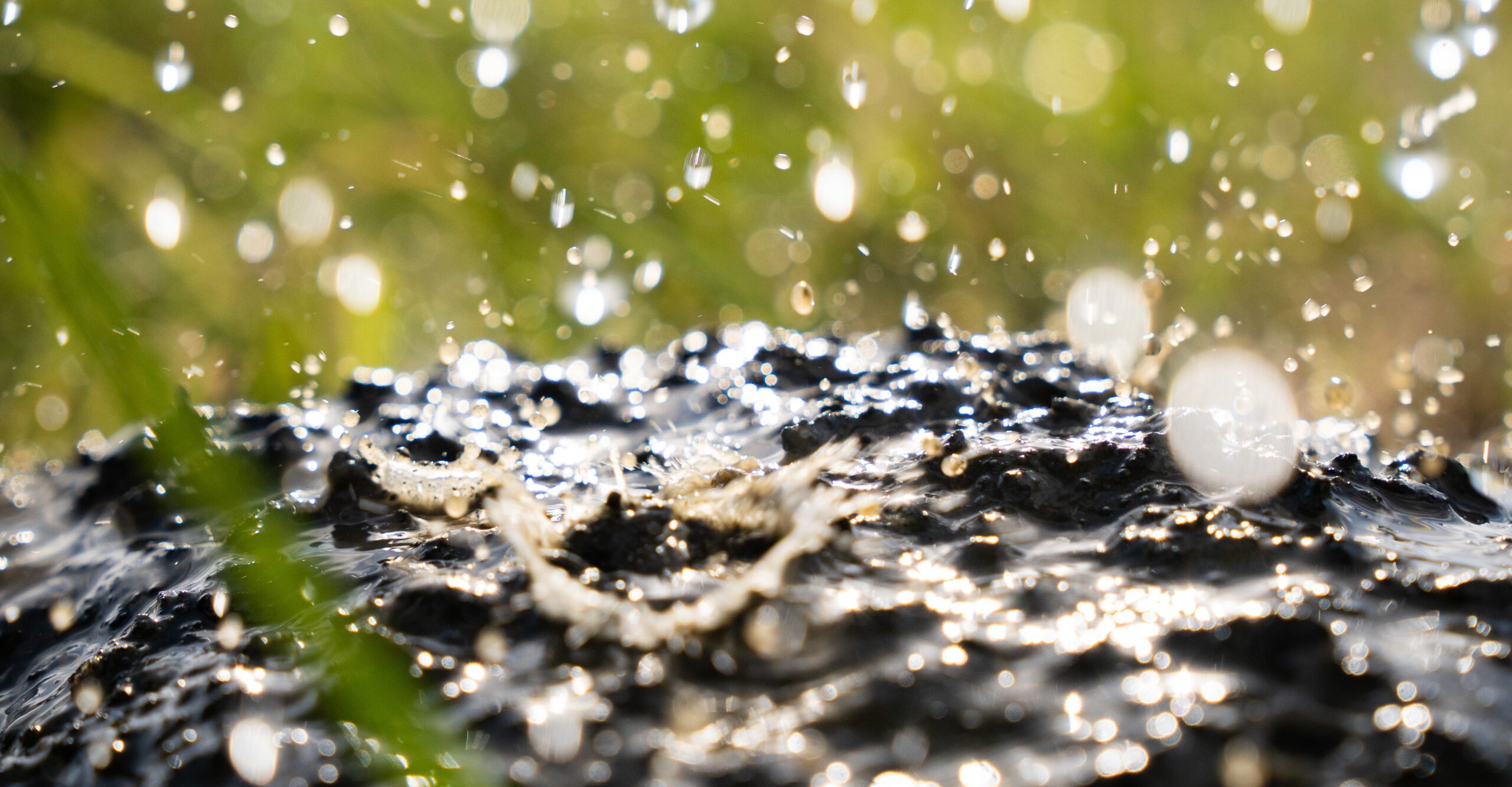This highly detailed and photorealistic close-up photograph captures raindrops falling and splashing onto a solid, jagged surface reminiscent of dark, wet, alligator skin. The lower half of the image showcases this textured ground in sharp focus, emphasizing the droplets as they hit and bounce upwards, creating a dynamic and lively scene. On the left side, a single blurry blade of grass cuts across the foreground, adding a touch of natural greenery. The upper half of the photograph transitions into a beautifully blurred background featuring variegated green foliage and hints of light browns, contributing to a glowing, luminous effect. The raindrops in this section appear as light flares, emphasizing the motion and atmosphere of a rainy day. The overall composition skillfully contrasts the sharpness of the ground and water with the soft, indistinct backdrop, creating a mesmerizing visual experience.